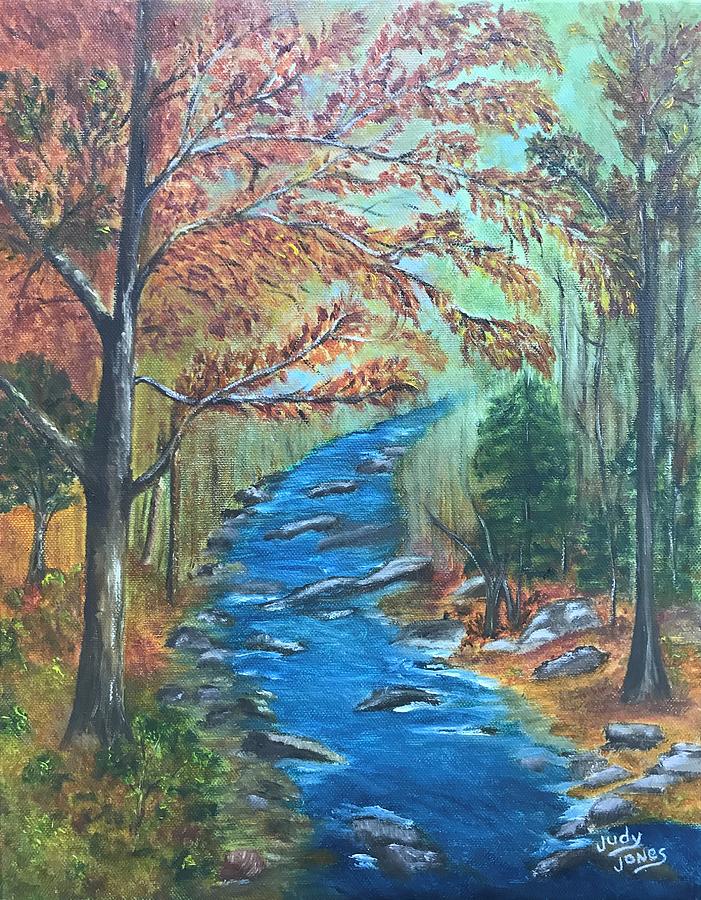This painting on canvas is a skillfully rendered woodland landscape by the artist Judy Jones, who has signed her name in white ink in the lower right corner of the artwork. The central feature of the painting is a vibrant, azure blue stream, dotted with black rocks that create a slight white taint where the water cascades over them. The stream winds its way from the lower right corner towards the middle of the painting, where it fades into the background. Flanking the stream on either side are dense forest scenes. 

On the left bank, a prominent tree with reddish-brown leaves, indicative of the fall season, stands out against a backdrop of smaller trees and patches of tall grass that recede into the background. Contrasting this, the right side of the stream features a slightly smaller but still large tree with greener foliage, suggesting it might be of a pine variety. The woodland to the right also includes smaller trees and rocks, adding to the varied texture of the landscape. The overall scene is bathed in bright, vivid hues that suggest a sunny day in late autumn, with a mix of orange, green, blue, and white colors contributing to the lively yet serene atmosphere depicted.